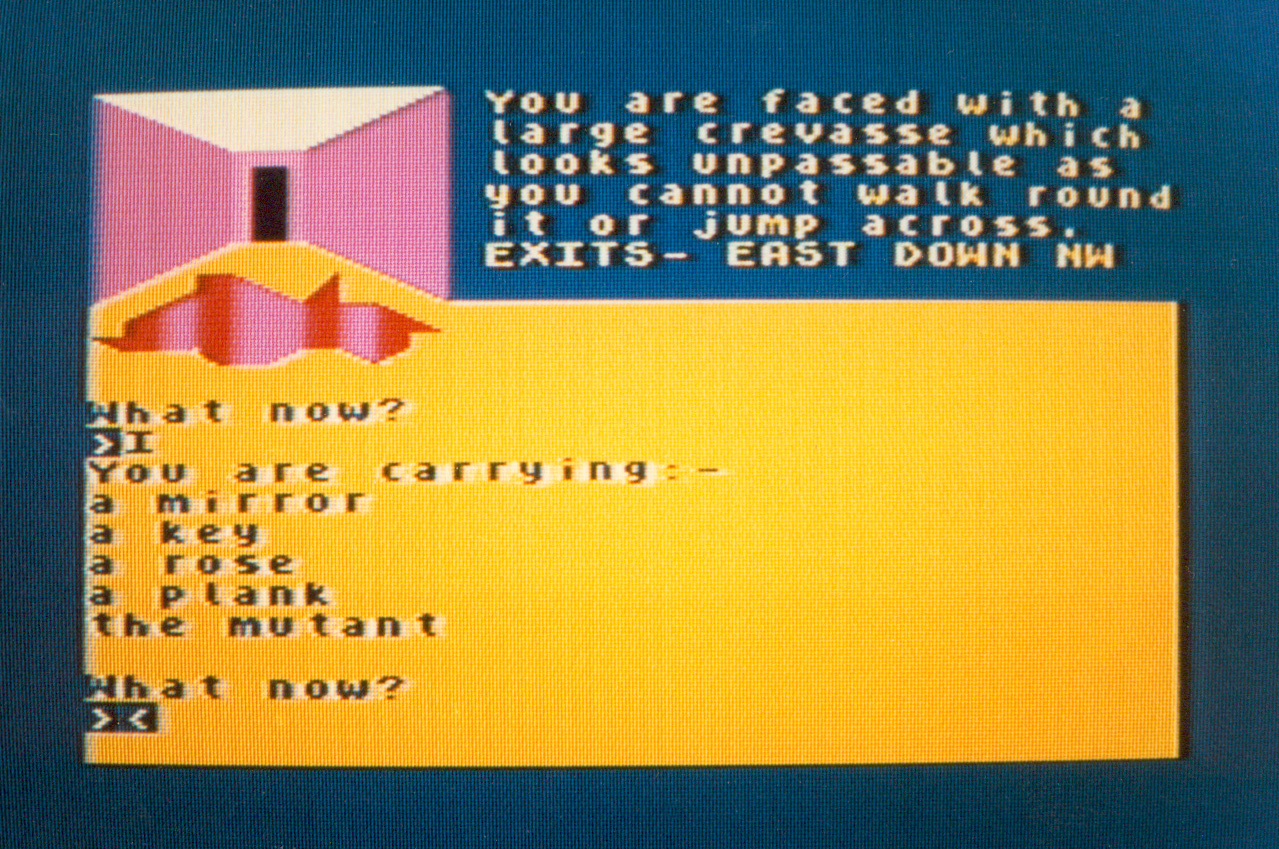We are looking at a pixelated screenshot from an old role-playing video game displayed on an antiquated computer monitor. The overall background of the screen is dark blue. Dominating the scene in the upper left corner is an image of a corridor characterized by pink walls, a white ceiling, and a black doorway at the end. In the center foreground of this hallway is a red object, which is revealed to be a deep crevice or hole in the game's narrative.

To the right of the corridor image, there is a yellow paragraph of text that reads: "You are faced with a large crevice which looks unpassable as you cannot walk around it or jump across. Exits east, down, northwest." Below this, a gold box with black font prompts the player with the question, "What now?" and lists the items the player is carrying: a mirror, a key, a rose, a plank, and the mutant. There are also two blue squares with arrows indicating interactive command inputs for the player's next action. The nostalgic aesthetic and simple graphics highlight it as a low-tech game compared to modern standards.